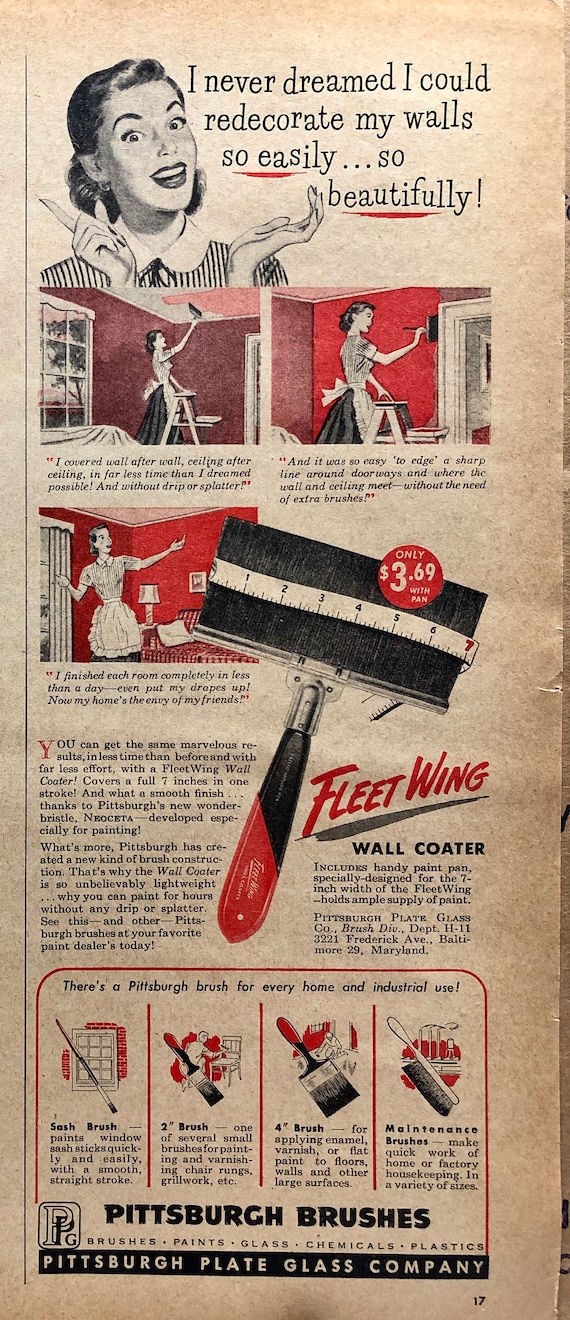This vintage advertisement from Pittsburgh Plate Glass Company features a black-and-white image with red accents, promoting their Fleet Wing Wall Coater. The ad, which looks as if it came from an old newspaper or magazine, showcases a 1950s housewife with an old-fashioned hairstyle and vibrant red lipstick, exclaiming, "I never dreamed I could redecorate my walls so easily, so beautifully."

In a series of three panels, the woman is shown redecorating her walls with ease: first, she's on a step stool painting the ceiling; next, painting around a door; and finally, admiring her finished room with satisfaction. Adjacent to these illustrations, there is a detailed image of the Fleet Wing Wall Coater, a brush that's seven inches wide, priced at only $3.69. The brush is depicted with a measuring tape to emphasize its width, and additional information about its features is provided.

At the bottom of the ad, it declares, "There's a Pittsburgh brush for every home and industrial use," and highlights four different brush types offered by the company. The advertisement rounds off with the Pittsburgh Plate Glass Company logo, stating their product range including brushes, paints, glass, chemicals, and plastics, all illustrated in a classic black-and-red color scheme.